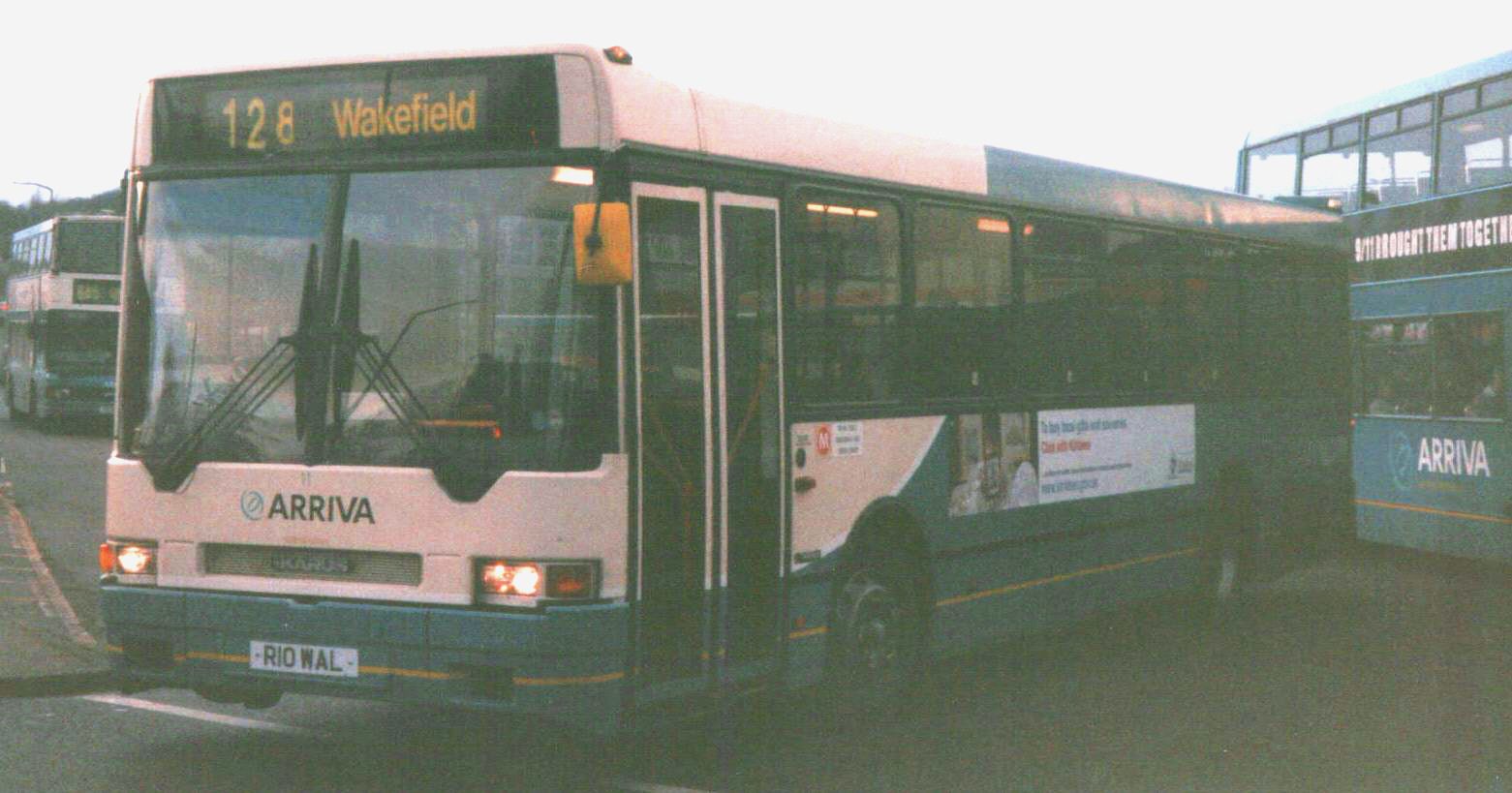The image depicts a somewhat hazy and aged scene featuring three Arriva buses, suggestive of either a bus parking or servicing area. The most prominent bus in the center bears a sign at the top displaying "128 Wakefield" in yellow text. This bus showcases a white and dark blue color scheme, with a defining yellow stripe along the base that encircles the entire vehicle. The front section of the bus includes a notable swoosh pattern that separates the white top from the blue bottom, and its headlights are on, illuminating the scene. Additionally, the bus has "Arriva" prominently displayed in capital letters on the front, accompanied by a license plate that reads "RIOWAL." Surrounding the main bus are two other double-decker buses of the same Arriva company, positioned on the left and right, both sharing similar blue and white hues. The setting appears to be a cemented area, under a light bluish-gray sky, contributing to the picture's overall dark and grainy appearance.